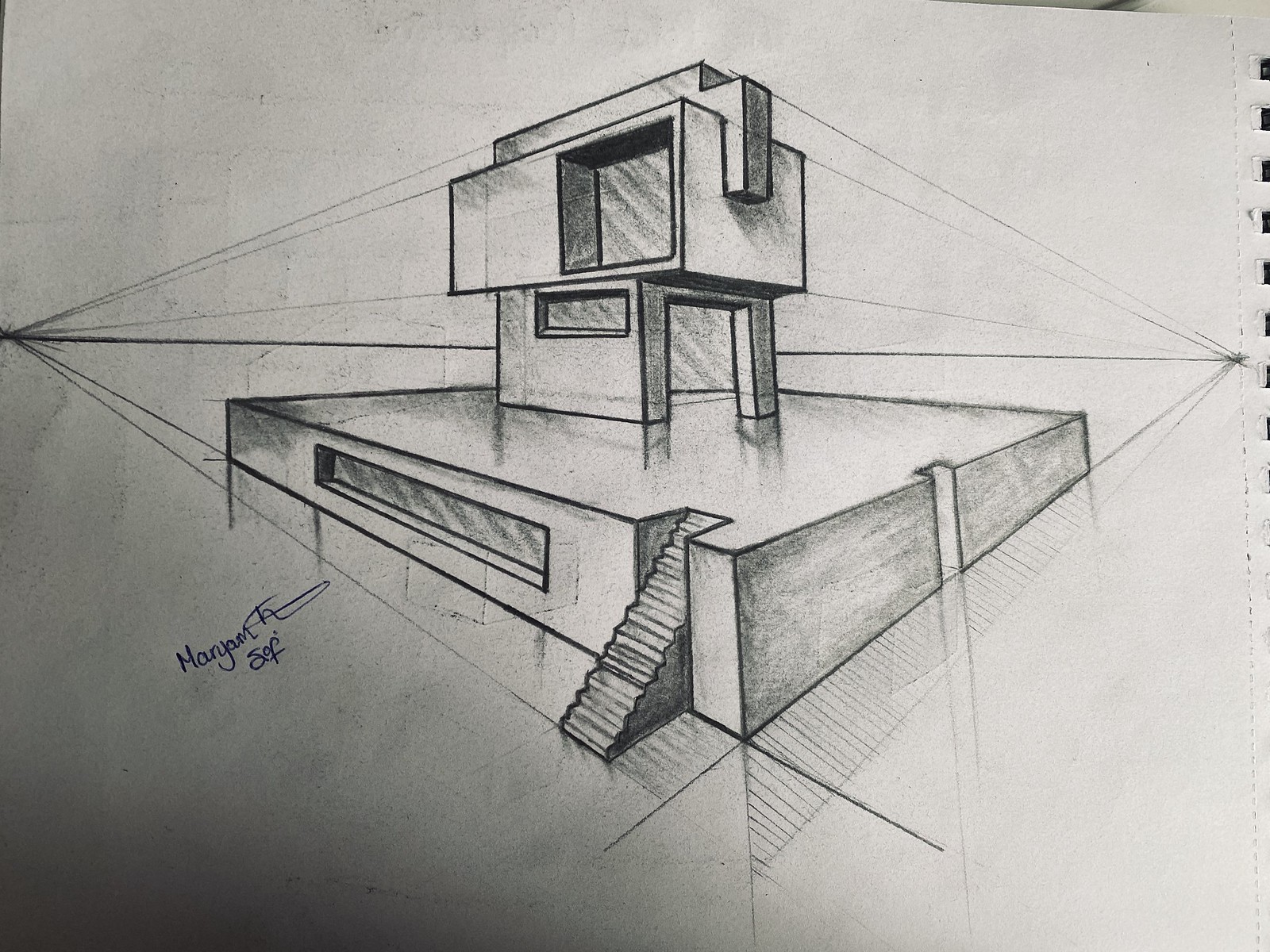The image is a highly detailed pencil or charcoal drawing of a geometrical, modern building concept, resembling a blend of retro and contemporary architectural styles. The composition is centered around a low rectangular platform featuring an exterior set of stairs on the right. A long horizontal window is prominently visible on this lower level. Above this platform, the building expands into two stacked box-like structures, each with distinct windows and doors. The lower box includes an open doorway and another elongated window. The upper level has a large, square window that appears to function like a slider. The scene is framed by radial lines originating from the left and right edges, converging towards the center. Additional details include a signature in blue ink reading "Maryam H" in the lower left-hand corner, and perforations along the right edge from being torn out of a notebook. The drawing is rendered on white sketching paper.